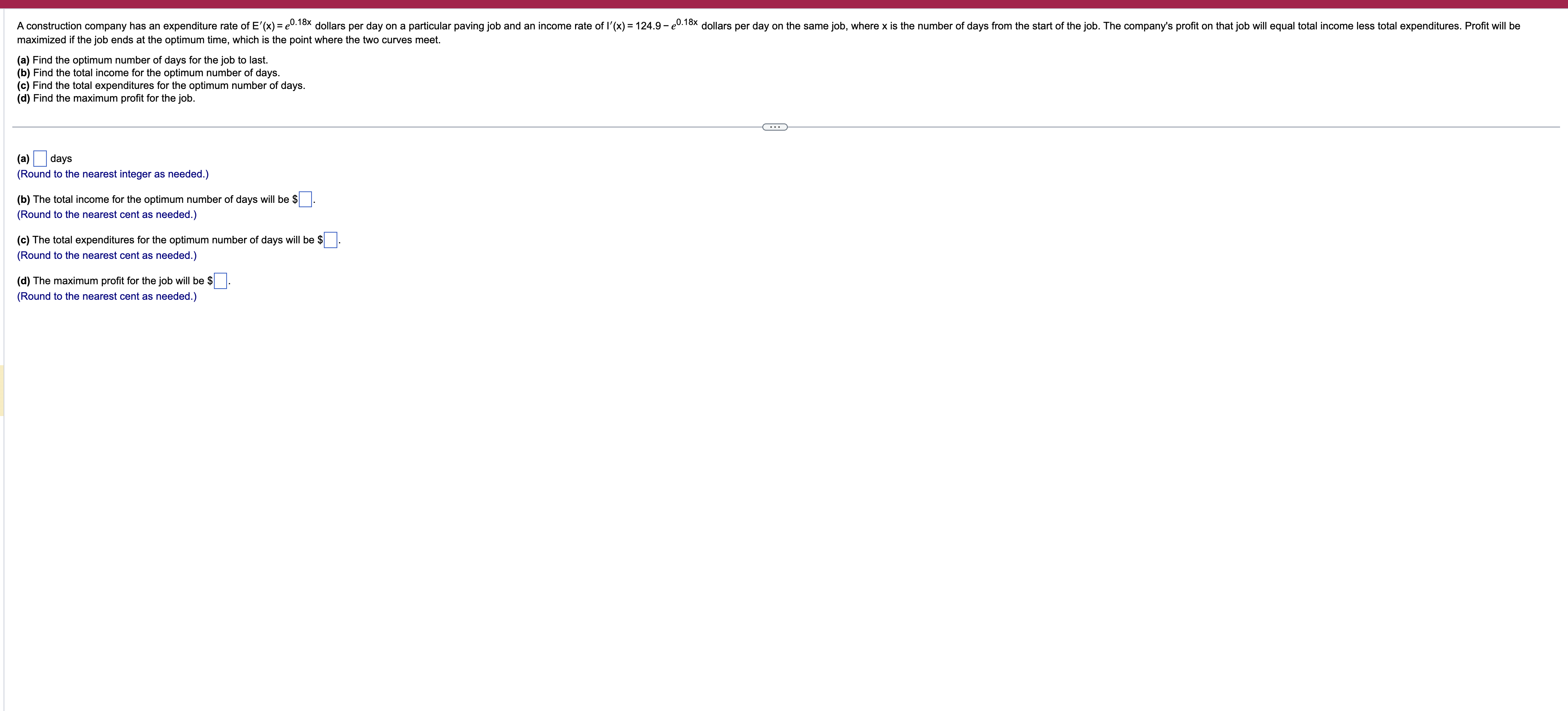The image depicts a webpage featuring a mathematical test question related to a construction company's expenditures and income rates.

**Caption:**

The webpage displays a red navigation bar at the top, beneath which there is a detailed test question presented in black text on a white background. The problem involves the expenditure rate, \( EX \), and income rate, \( LX \), of a construction company. Specifically, their expenditure rate per day is given by the function \( EX = e^{0.18X} \) dollars, while their income rate per day is \( LX = 1.249 - e^{0X18} \) dollars, where \( X \) represents the number of days since the start of the job. The task is to determine at what point the job should end to maximize profit, which occurs where the expenditure and income curves intersect.

The question asks for several calculations:
A. Determine the optimal number of days the job should last.
B. Calculate the total income for those optimal days.
C. Compute the total expenditures over the optimal number of days.
D. Find the maximum profit the company can achieve on the job.

Additionally, response fields labeled A, B, C, and D are provided to answer these sub-questions, with instructions to round numbers to the nearest integer as needed. The text acknowledges the algebraic nature of the question, indicating a challenge for those less confident in algebra.

In summary, the webpage is solely dedicated to this test question concerning the optimal completion time for a job to maximize the construction company's profit.